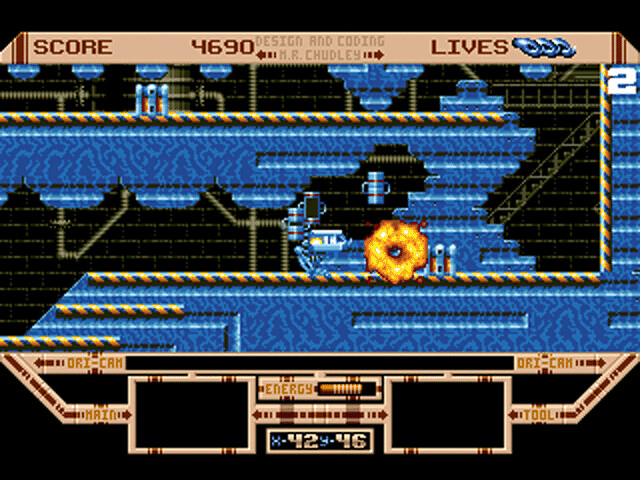This image captures a retro video game screen with a minimalist design. At the top, the score is displayed as "4690" alongside the text "Design and Coding by Mr. Chudley". The screen also indicates the player's lives with three small blue creatures. The background features blue metal ramps with a notable yellow, donut-sized fireball situated on the bottom ramp. Beneath these ramps, an additional section provides further information, showing labels such as "Dry Cam Main," "Energy," "Dry Cam Tool," and numerical values "X 42, Y 46" for additional scoring or game metrics. The blue ramps and text stand out vividly against the stark black background, creating a striking contrast that emphasizes the game's simplicity and design elements.